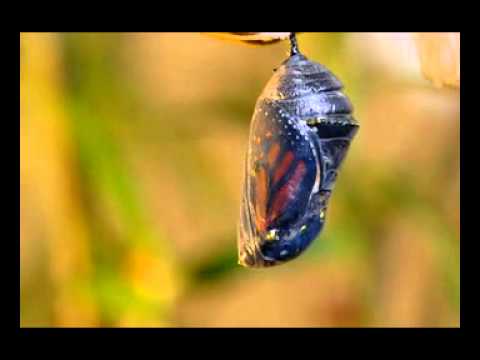This highly detailed nature photograph captures the intricate beauty of a monarch butterfly chrysalis in the wild, moments before it emerges. The chrysalis hangs upside down, its dark, shiny casing tapering into a cylindrical shape with a smoother left side and more ribbed, indented right side. A see-through area reveals the vibrant wing pattern of the monarch butterfly inside, showcasing shades of orange with black edges, signaling its imminent emergence. The blurred background enhances the subject, featuring a blend of yellow, light green, and dark green hues. The open air around the chrysalis adds to the anticipation of the transformation about to unfold, emphasizing nature's delicate and mesmerizing process.